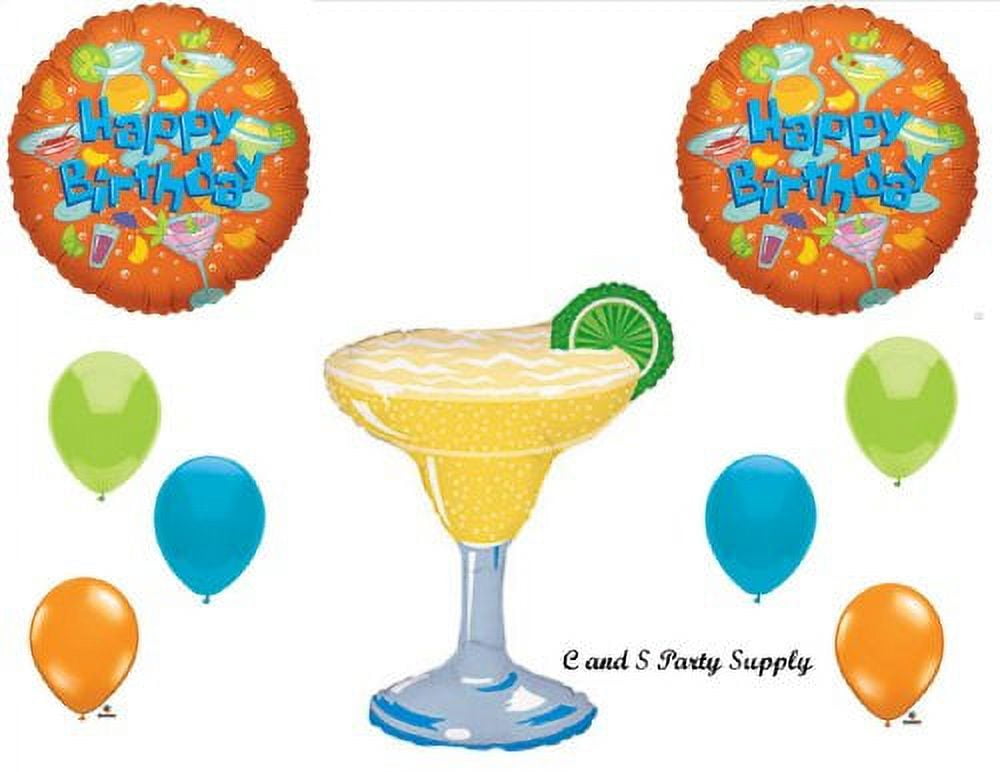This vibrant and festive digital artwork showcases an assortment of cartoon-styled party supplies with a central focus on a margarita theme. At the heart of the image lies a detailed margarita glass, filled with a golden-yellow drink and garnished with a round lime slice on the rim. Surrounding the glass, on both the left and right sides, are clusters of three colorful balloons—green, blue, and orange—arranged in a mirrored pattern.

Prominent at the top corners of the image are two identical orange foil balloons, each emblazoned with "Happy Birthday" in bright blue letters. These balloons feature an array of cocktail illustrations, including margaritas, daiquiris, and other drinks, accompanied by lemon and lime slices, lending a lively and celebratory ambiance to the design.

Though the overall background of the image is plain, a subtle design detail includes a thin gray line forming a partial top border. Additionally, in the bottom right corner, "CNS Party Supply" is clearly printed in black letters, branding the festive scene. The cohesive use of bright colors and playful elements encapsulates a jubilant atmosphere perfect for any birthday celebration.